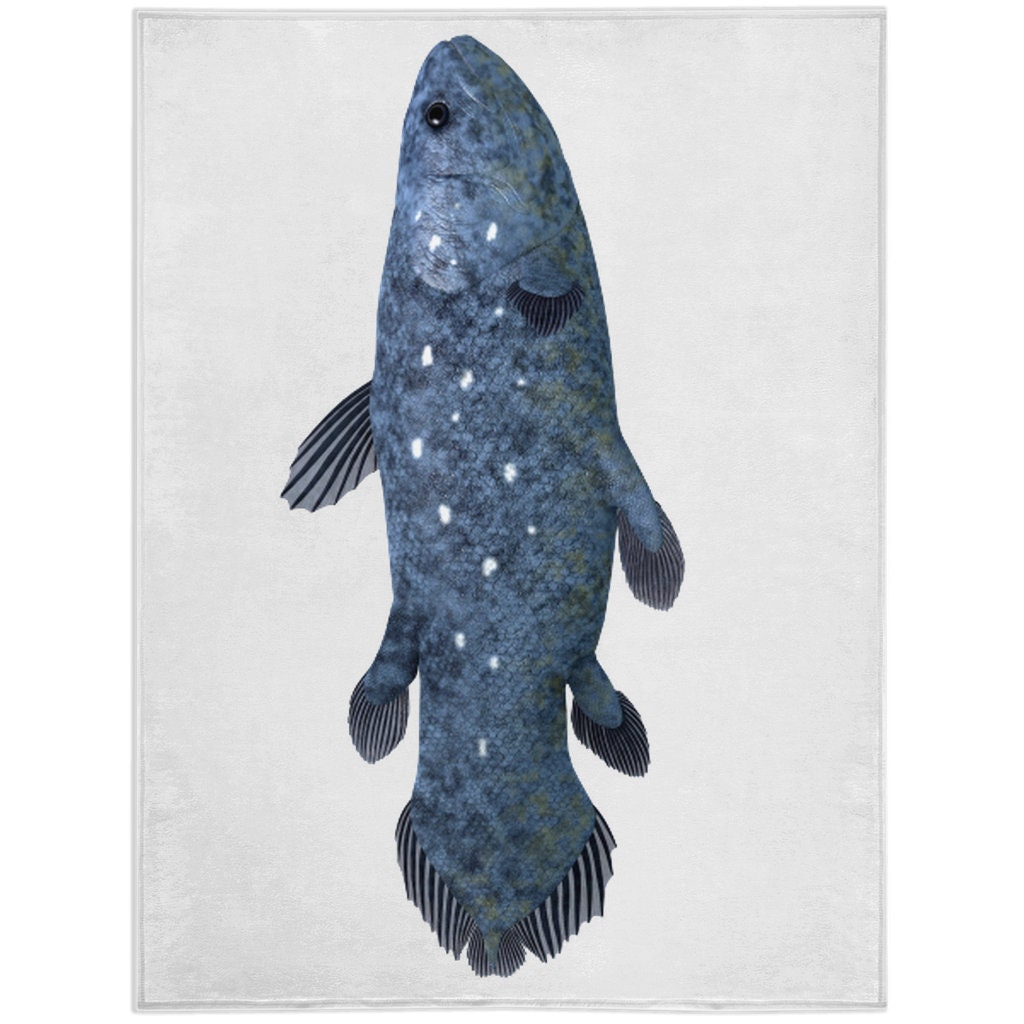The image depicts a side-view artwork of a fish, set against a pale white, portrait-oriented canvas. The fish is positioned with its head at the top and its tail at the bottom. The body of the fish is rendered in various shades of blue and gray, with white specks scattered along its side, possibly representing light reflection or light-colored scales. The fins are detailed with black and gray stripes, adding to the intricate appearance. The fish's scales, gills, eye, and mouth are all clearly visible, emphasizing the detailed artistic representation. The nature of the artwork makes it ambiguous whether it is a realistic depiction of a natural fish, a painted piece, or even an AI-generated image, but it distinctly showcases the artist's attention to fine details and coloration.